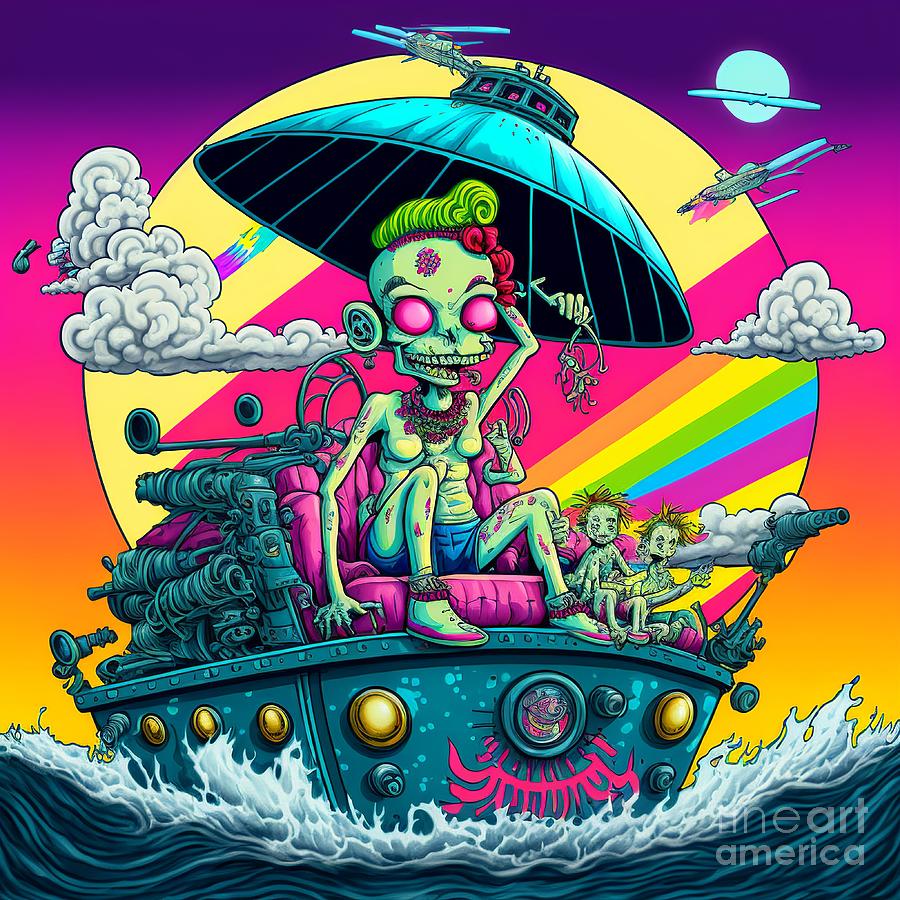This vibrant New Age-style art piece bursts with an array of bright colors, creating a striking visual impact. The background transitions from dark purples at the top, descending through gradients of pink, peach, orange, and culminating in yellow, while the bottom half depicts a deep blue ocean with white waves. Central to the artwork is a metal boat gliding across the sea; its bluish-green hull adorned with gold circles evenly spaced about an inch apart, and two additional gold circles on the stern. At the heart of the stern is a circular emblem featuring an alien-like figure with a pink design radiating from its center.

Seated prominently at the front of the boat is a skeletal figure with pale skin and tattoos. Its distinctive appearance includes large pink eyes, a green mohawk with pink tips, and a lean physique. Dressed in blue jean shorts, white shoes accented with a pink stripe, and a tank top, the skeleton also wears a colorful lei around its neck. This figure sits in a bright pink chair evocative of a throne amidst its peculiar crew—two smaller, grass-like figures resembling children flanking it.

Behind the central figure, a large, golden sun with rainbow-hued lines emanates vibrantly, adding to the sense of otherworldly illumination. On the left side, a soft cloud adds a contrasting touch to the otherwise intense color palette. At the bottom right of the image is the artist's signature or title, "The Art America," anchoring this detailed, imaginative scene that melds elements of steampunk, fantasy, and surrealism.